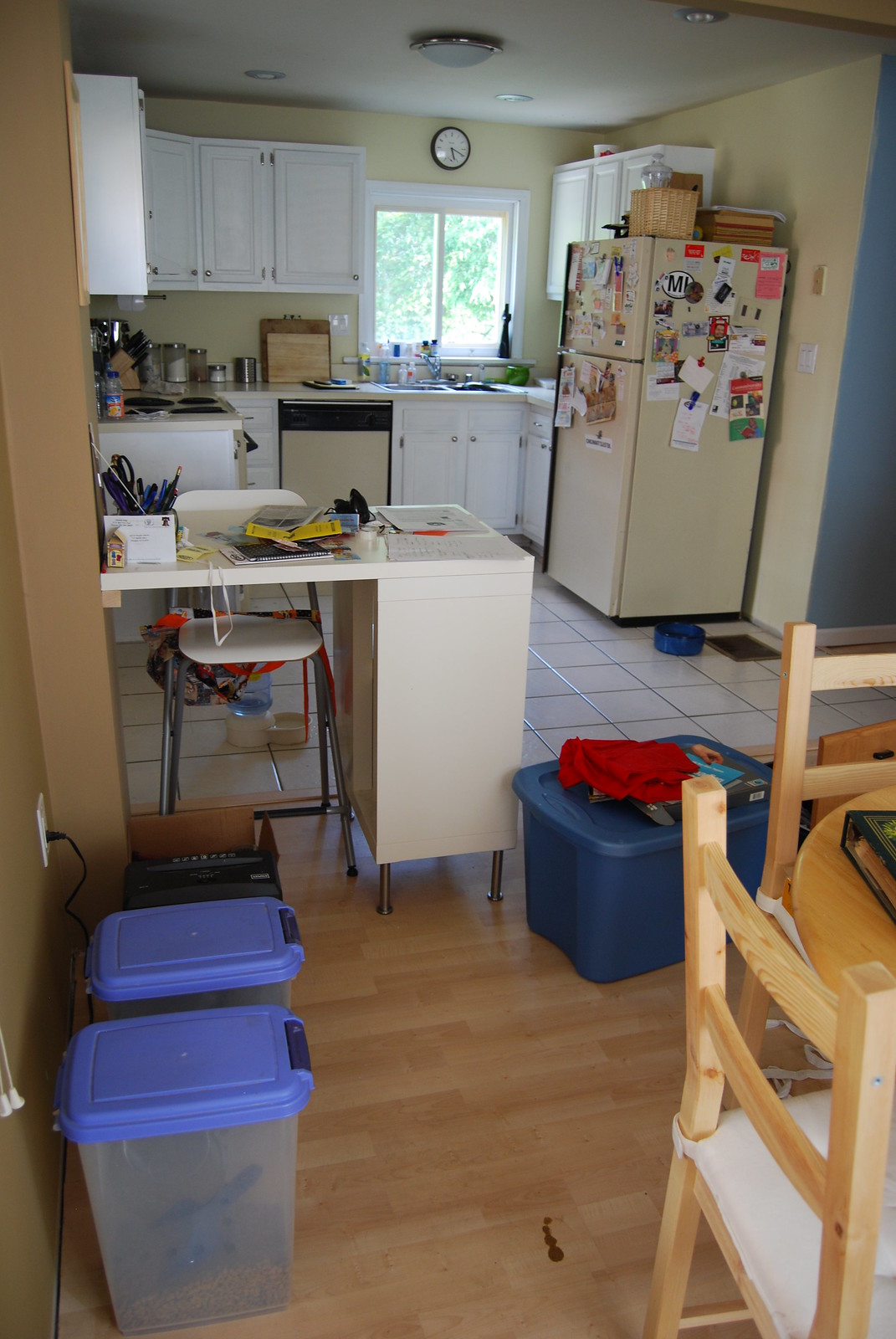This image captures a cluttered kitchen showcasing a mix of wooden and white tile flooring. The walls are painted in various colors, transitioning from brown to off-white in the kitchen, with a blue hallway in the background, creating a vibrant and somewhat eclectic atmosphere. The refrigerator is adorned with numerous clippings, photos, stickers, and magnets, and is topped with additional clutter. White cabinets frame a window above the sink, which sports a clock reading 5:20. The off-white dishwasher and fridge blend seamlessly with the kitchen walls. On the countertop, a collection of cutting boards, spices, flour, and a knife set surround the stove.

Closer to the foreground, a cluttered white midsection desk bridges the kitchen and living room, scattered with notebooks, pens, a stapler, and other miscellaneous items. Beneath the desk sits a paper shredder, alongside two Rubbermaid containers filled with dog food, each containing a scoop. A spill of an unknown brown substance stains the floor nearby. In the bottom right corner of the image, the edge of a table is barely visible, completing the scene of this busy and lived-in kitchen space.